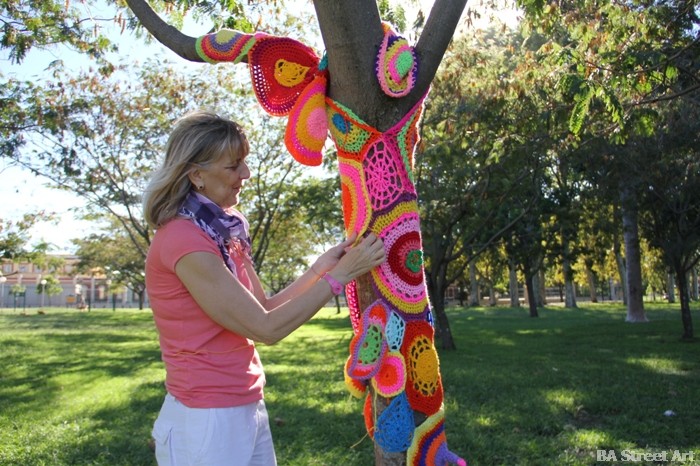In this vibrant city park on a bright, sunny day, an older white woman with blonde hair is engaging in a unique street art project. She stands near the middle left of the image, wearing a purple scarf, a pink top, and white slacks. Against a backdrop of beautiful green grass, numerous trees, and a distant building on the far left, she meticulously wraps and connects an array of multicolored, crocheted doilies around the trunk of a large tree. These intricate, handmade doilies, featuring a variety of patterns including circles and webs, showcase an explosion of colors—ranging from purple, red, green to yellow, pink, and light red. Her artistic endeavor is seemingly part of a street art installation, as indicated by the "BA Street Art" inscription in the bottom right corner. The morning sky is a clear, bright blue, accentuating the lively and creative atmosphere of the scene.